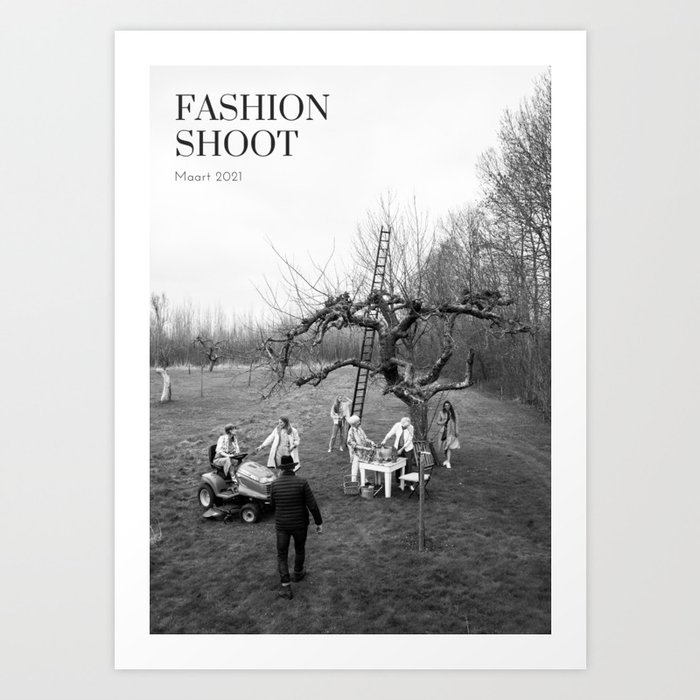The cover of the magazine "Fashion Shoot," dated March 2021 (Maart 2021), features a striking black-and-white photograph bordered in white. This detailed scene, filled with a sense of timeless human activity, captures a group of people gathered around a large, leafless, gnarly tree in a field. To the left, a person is riding a lawnmower and conversing with another individual, who is dressed in a black hat and a dark outfit, possibly a fedora and puffer jacket. Walking toward them is another person in a long coat. 

Central to the photograph is the dead tree itself, with a tall bamboo ladder propped against one of its bare branches, suggesting a potential climb. Beneath the tree, there is a table setup. Two older women are engaged at the table, which has various items that could be work supplies or picnic materials, along with empty baskets. Three tall, thin women with long hair, wearing long coats, are also present in the scene. One woman, possibly holding a microphone, seems to be reporting. The setting is framed by other winter-bare trees at the perimeter of the field.

The overall ambiance of the photograph is one of a collaborative effort or candid moment amidst nature, beautifully encapsulated in the monochromatic palette of the image.